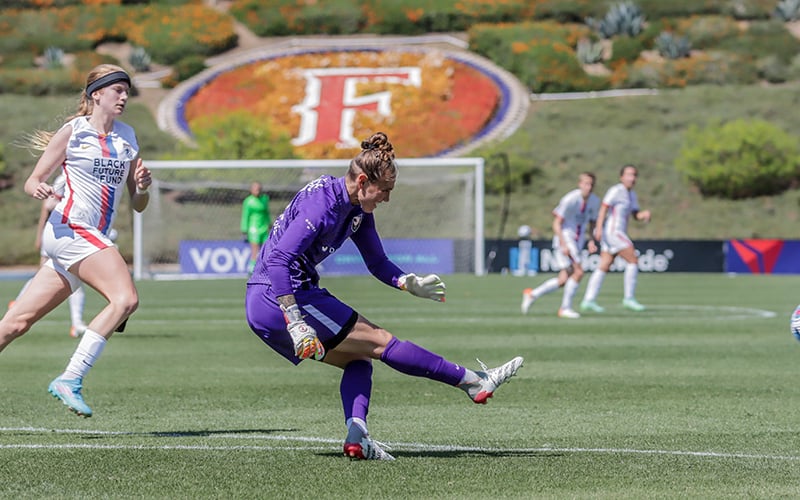In this vividly captured photograph of a co-ed soccer game, the central focus is a woman dressed in a deep purple uniform with a white stripe down the side. She has just kicked the ball and is featured mid-motion with her leg still in the air. Her attire includes long purple socks that reach up to her knees, white gloves, and white cleats featuring orange accents. Her hair is styled in a bun with an undercut.

Directly behind her, an opposing team member is seen sprinting towards the ball. This woman is clad in a white uniform adorned with red and blue stripes down the front. Her outfit also includes mid-calf white soccer socks and aquamarine cleats. She sports a black headband that holds back her long blonde hair, tied in a ponytail braid. The white jersey also features the Nike logo and the text "Black Future Fund."

In the distance, two male players, intently focused on the ball's trajectory, are positioned to either intercept or follow its path. The game is being played on a pale green turf, possibly in a college stadium, indicated by the large letter 'F' on the lawn outside the arena. The photograph is set in broad daylight, adding clarity and vibrance to the dynamic scene.